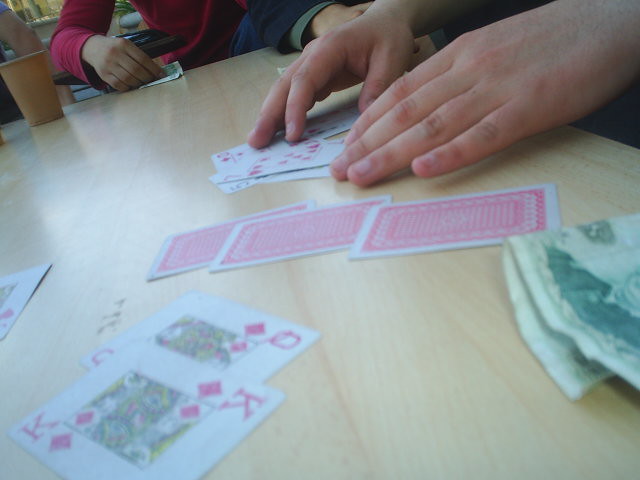The photograph captures an intimate and detailed moment at a card game, focusing on a close-up of the table where two individuals are engaged in play. The scene is slightly faded, perhaps indicative of a photograph taken with a point-and-shoot camera, and it is rendered in full color.

In the bottom-left corner, two face-up cards draw immediate attention: a King of Diamonds prominently displayed with a Queen of Diamonds peeking out from behind. Just above these cards, three more cards lie face-down in a neat, slightly overlapping row, hinting at the mystery of the game in progress.

To the right side of the image, a folded piece of currency subtly suggests a potential wager or an added layer of stakes to the game. 

Above the face-down cards, a pair of hands are actively engaged with a spread of face-up cards on the table, implying a moment of critical decision-making or reshuffling. This intimate hand action adds a sense of movement and engagement to the scene, making one ponder the dynamics and strategies at play.